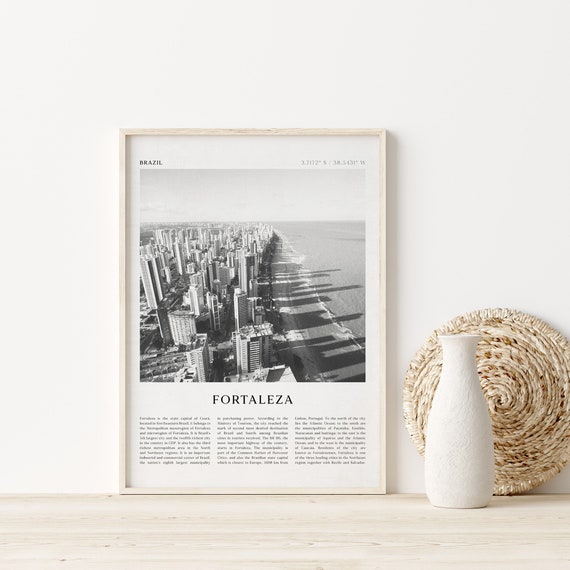The photograph showcases a neatly arranged setting featuring a large framed poster leaning against a pristine white wall atop a bleached white wood tabletop. To the right of the poster sits a small white milk bottle, flanked further in the background by a round, woven raffia placemat. The poster, outlined in an off-white wooden frame, prominently displays the word “Fortaleza” beneath a black and white aerial photograph of a beachfront cityscape, revealing towering skyscrapers closely lining the beach adjacent to the ocean. The top left corner of the poster reads “Brazil,” and the opposite corner lists compass coordinates, suggesting the location is Fortaleza, Brazil. Below the image are three paragraphs of tiny, nearly illegible text. The entire scene appears meticulously staged, imparting a clean and modern aesthetic.